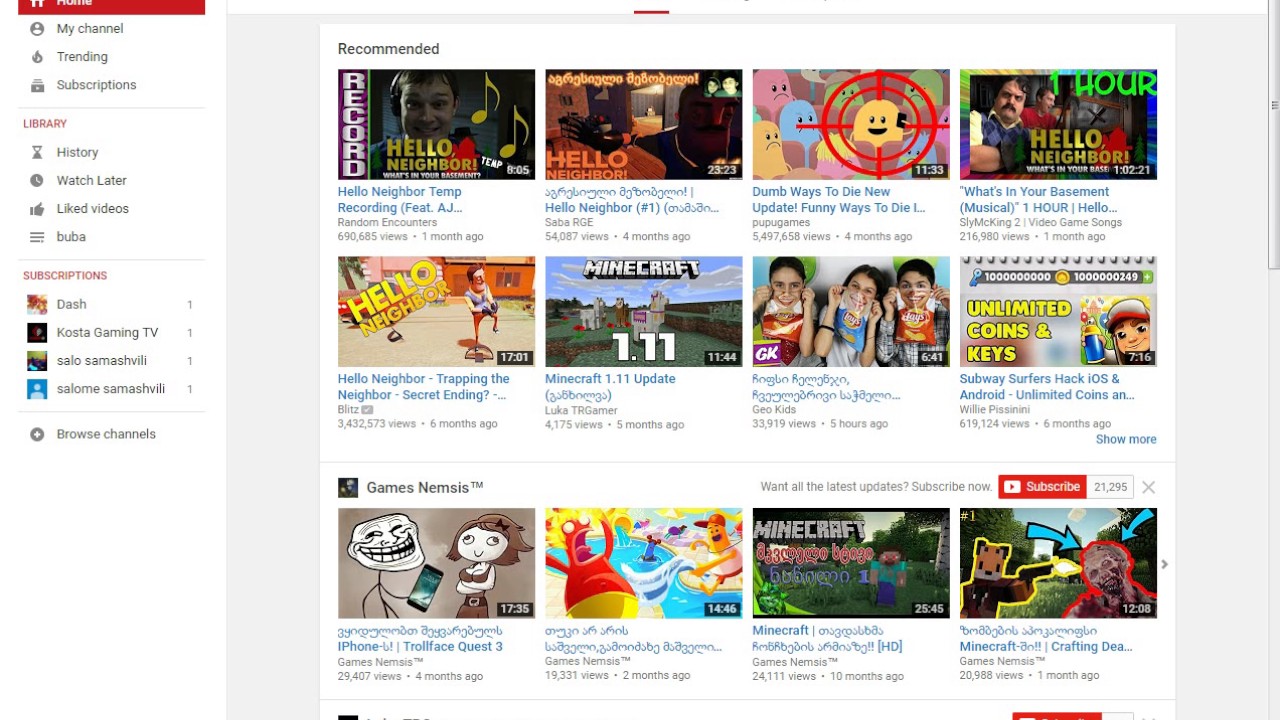The image depicts a web page interface, likely from a YouTube-like platform. On the left, there's a partially visible vertical menu displaying several navigation options including "Home," "My Channel," "Trending," "Subscriptions," "Library," "History," and "Watch Later." Some familiar icons and labels are visible, such as "Liked Videos" and a three-line menu icon labeled "Bubba." Below these, the "Subscriptions" section lists various channels such as "Cost a Gaming TV," "Say Low Semi," and "Salome Nashville," followed by a circular plus symbol labeled "Browse Channels."

On the right, the main content area is organized into three distinct rows of video thumbnails, each row having four thumbnails. The first row features:
1. "Hello Neighbor Temp Recording"
2. "Hello Neighbor"
3. "Dumb Ways to Die: New Update – Funny Ways to Die"
4. "What's in Your Basement Musical – One Hour"

The second row includes:
1. "Hello Neighbor Trapping the Neighbor"
2. "Minecraft 1.11 Update"
3. An unclear video featuring three kids with potato chips, titled by "Geo Kids"
4. "Unlimited Coins and Keys Subway Surfer Hack iOS and Android"

The third row contains:
1. "iPhone Troll Face Quest 3"
2. A video by "Games Nemesis" with cartoon characters screaming
3. Another "Minecraft" video by "Games Nemesis"
4. A third "Minecraft" video also by "Games Nemesis"

This detailed layout suggests a curated selection of recommended videos based on previous views or subscriptions, mixing gaming content with other entertainment genres.